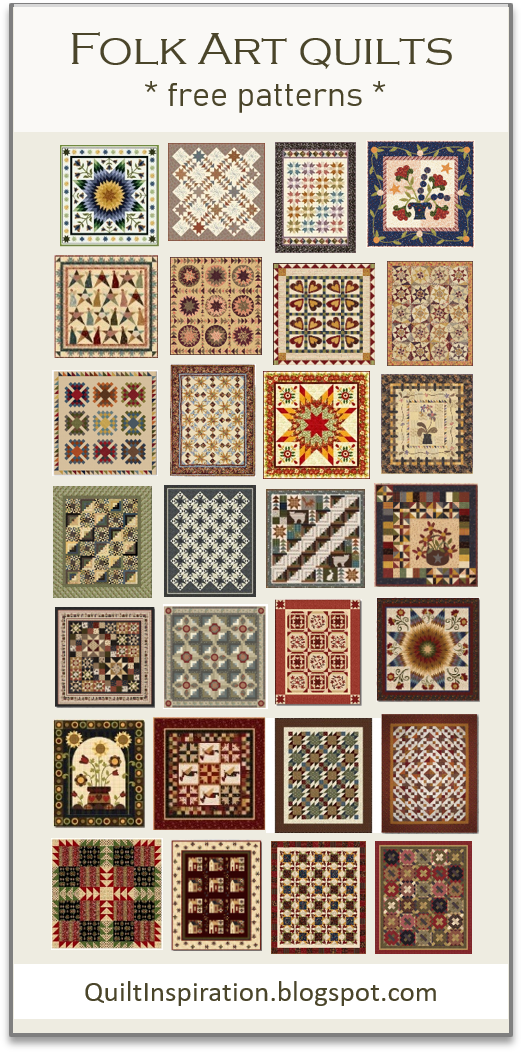The image is a vertically-oriented rectangular banner approximately two and a half to three times as tall as it is wide. The background is a muted off-white color. At the top of the banner, in black text, it reads "Folk Art Quilts" followed by "Free Patterns." Below this text, spanning the remainder of the banner, is a grid composed of four columns and seven rows, featuring a total of 28 different quilt designs. 

The quilt patterns are primarily in earthy tones—browns, greens, and reds dominate, with some accents of muted blues, light yellows, and oranges forming a predominantly pastel color palette. Many of the quilt designs feature recurring themes such as starbursts radiating from the center and regular grid patterns with varied colors.

At the very bottom of the banner, a white strip of text indicates the source website: "quiltinspiration.blogspot.com." The colors used for all text elements on the banner are consistently in shades of brownish-gray, harmonizing with the overall color scheme of the quilt designs.